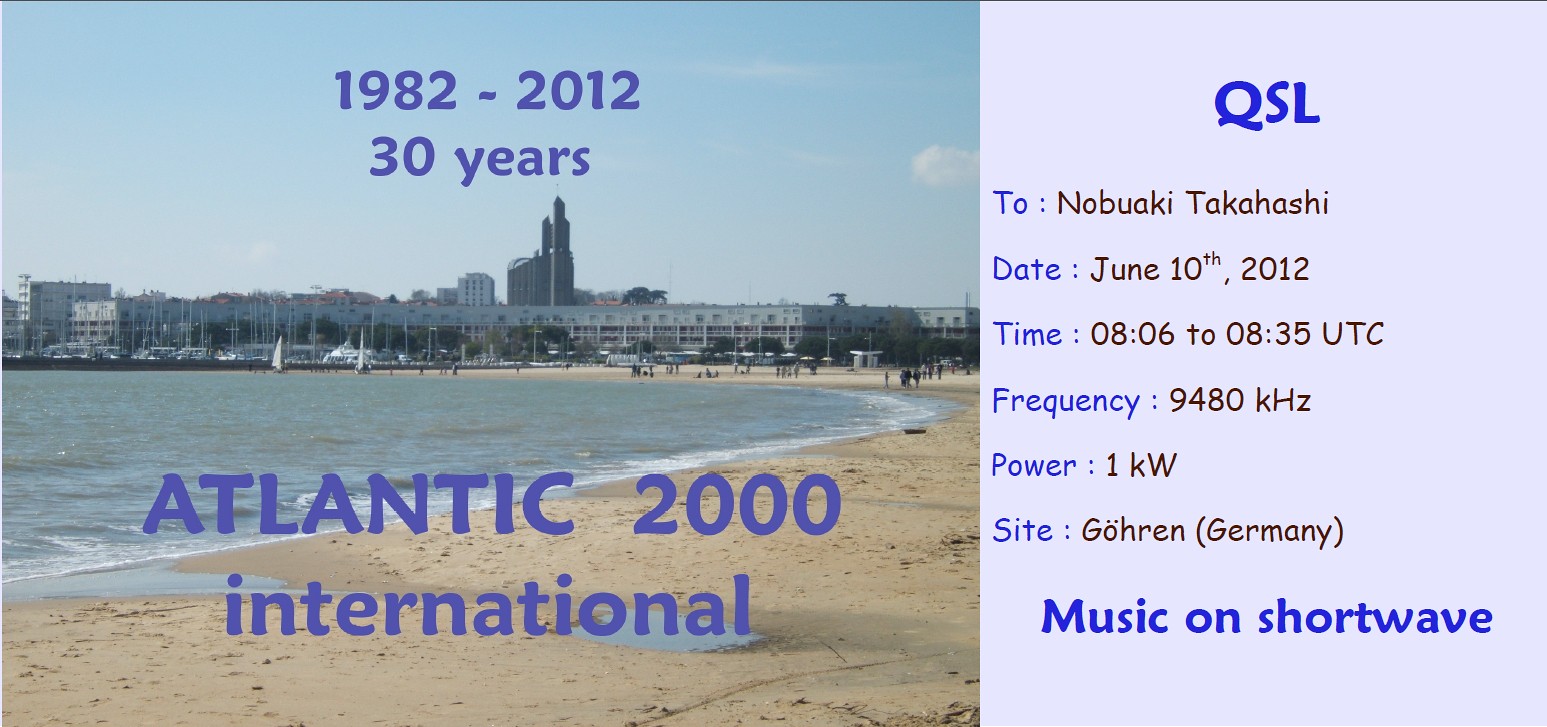The image is a photograph of a beach scene featuring the ocean with waves crashing onto the sand in the foreground. In the distance, on the right-hand side, there are several people walking along the shoreline. The background reveals a city skyline with buildings, possibly a bridge or a building with many windows, and several boats docked in the water. The sky is blue, becoming progressively hazy towards the horizon. 

Text overlaying the image in purple letters reads, "1982 to 2012, 30 years, Atlantic 2000 International." Along the right side of the photograph, a purple-bordered card contains detailed information: "QSL to Nobuaki Takahashi, date June 10, 2012, time 08:06 to 08:35 UTC, frequency 9480 kHz, power 1 kW, site Goren, Germany, music on shortwave." The palette includes blues, tans, greens, and purples, giving the overall appearance of a commemorative postcard from a radio station.